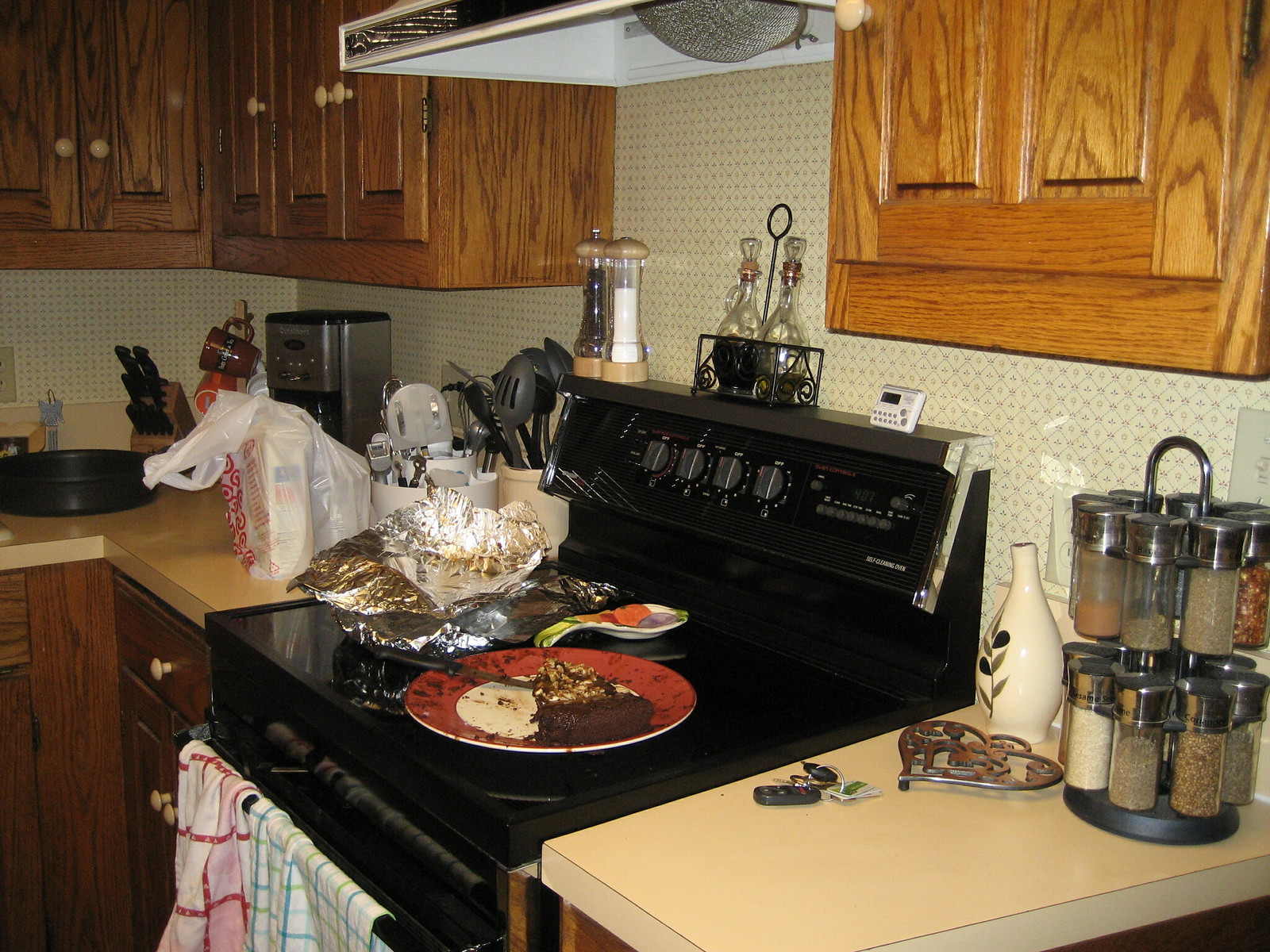A cozy 1970s kitchen scene is captured in this landscape image. The focal point is a classic black stove, adorned with a plate of food, a spoon rest, and remnants of foil likely used for cooking. Twin dish towels hang neatly from the stove's front rail. To the left, a tan coffee maker sits on the speckled countertop next to a bag of groceries and a coffee cup holder displaying several cups. In the corner, a knife block with an assortment of knives is paired with a black pan positioned in front. The right side of the stove features a narrow countertop holding a spice rack, a bottle of olive oil, a trivet, and a set of car keys. The kitchen's oak cabinets, fitted with white handles, complement the vintage aesthetic, and a ventilation hood hovers above the stove, ready to manage the day's cooking adventures.